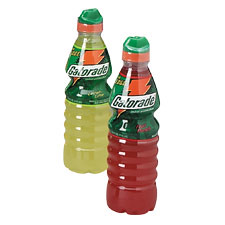This image features two bottles of Gatorade positioned side by side against a plain white background. The bottles are of the long and narrow variety, with a segmented design near the bottom that tapers as it ascends to the green and orange-striped sports caps. The bottle in the background is positioned slightly to the left and contains yellow Lemon-Lime Gatorade, while the bottle in the foreground is slightly to the right and holds red Fruit Punch Gatorade. Both bottles prominently display the Gatorade label on their upper halves, which is green with an orange lightning bolt superimposed on it. The lower halves of the bottles are clear, revealing the vibrant colors of the sports drinks within.